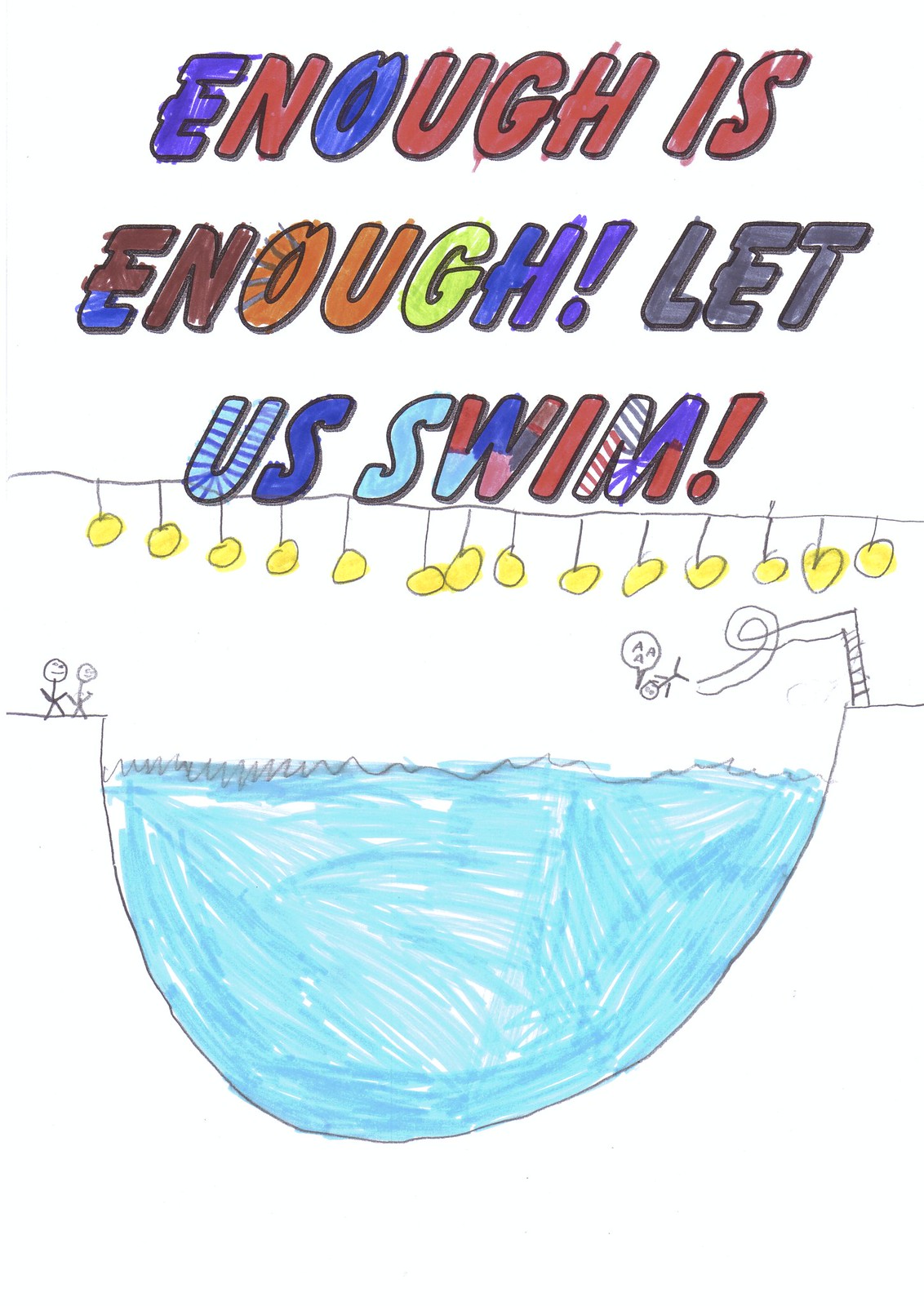This image is a child-like drawing of a swimming pool scene at the bottom, featuring a U-shaped pool filled with aqua-colored water. The pool is outlined in blue with a jagged black wavy line at the top, giving the impression of water splashing. There are five stick figures depicted: two standing to the left and one on the right diving off a diving board into the pool, exclaiming, "Ah, a-a-a" in a speech bubble. Above the pool, a series of about 15 yellow lights hang on stems extending from a horizontal line. The top of the drawing features the text, "Enough is enough! Let us swim!" in a variety of colors, including blue, red, orange, brown, and green. The letters appear to be colored in with markers, but the coloring goes outside the lines, suggesting it was done by a child.